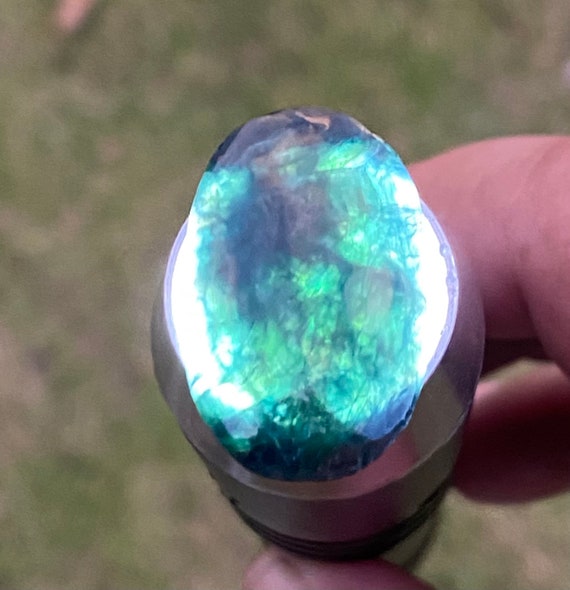The image is a close-up shot of a hand holding an oval-shaped, precious stone that occupies the majority of the frame. The stone, which resembles both jade and a glowing gem, features a dynamic mix of colors — predominantly green with hints of dark blue, purple, and opalescent pearl-like reflections. It rests on a small, round brown platform, detail that complements the intricate, brain-like patterns within the stone, which is characterized by its green crystalline center and dark blue edges. The background is a blurred grassy field, with the focus sharply on the hand and the stone, highlighting the stone's unique beauty and fine craftsmanship.